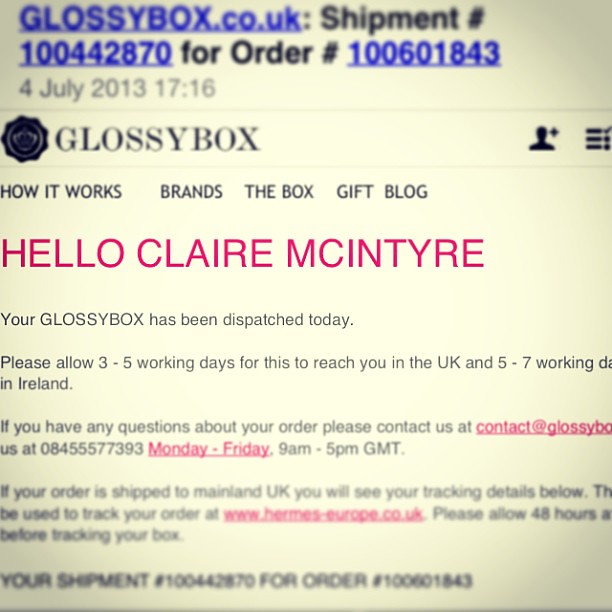The image is a large, slightly blurry square, particularly at the top and bottom. At the top, it displays "Glossybox.co.uk" in blue, followed by a shipment number "10442870," and the date "4 July 2013 17:16". Below, a subtle grey line separates this information from a black circular logo with "Glossybox" in all caps next to it. Another grey line delineates the logo from a series of headings: "How It Works," "Brands," "The Box," "Gift," and "Blog." On the right, there's an icon representing a person's silhouette with a drop-down menu, typical of user account interfaces on websites.

The email text begins under these headings with a warm greeting in large pink all-caps: "HELLO CLAIRE MCINTYRE." Following in left-aligned black text, it reads, "Your Glossybox has been dispatched today. Please allow 3-5 working days for this to reach you in the UK and 5-7 working days in Ireland." An additional instructional line says, "If you have any questions about your order, please contact us at contact@Glossybox.com. Our phone lines are open Monday through Friday, 9 to 5 pm." This section is somewhat blurred, making some details hard to read. The email continues, "If your order is shipped to mainland UK, you will see your tracking details below. Please allow 48 hours before tracking your box." At the bottom, it repeats the shipment number for the order, which is also somewhat blurry. Overall, the image appears to be a screenshot of an email from Glossybox.